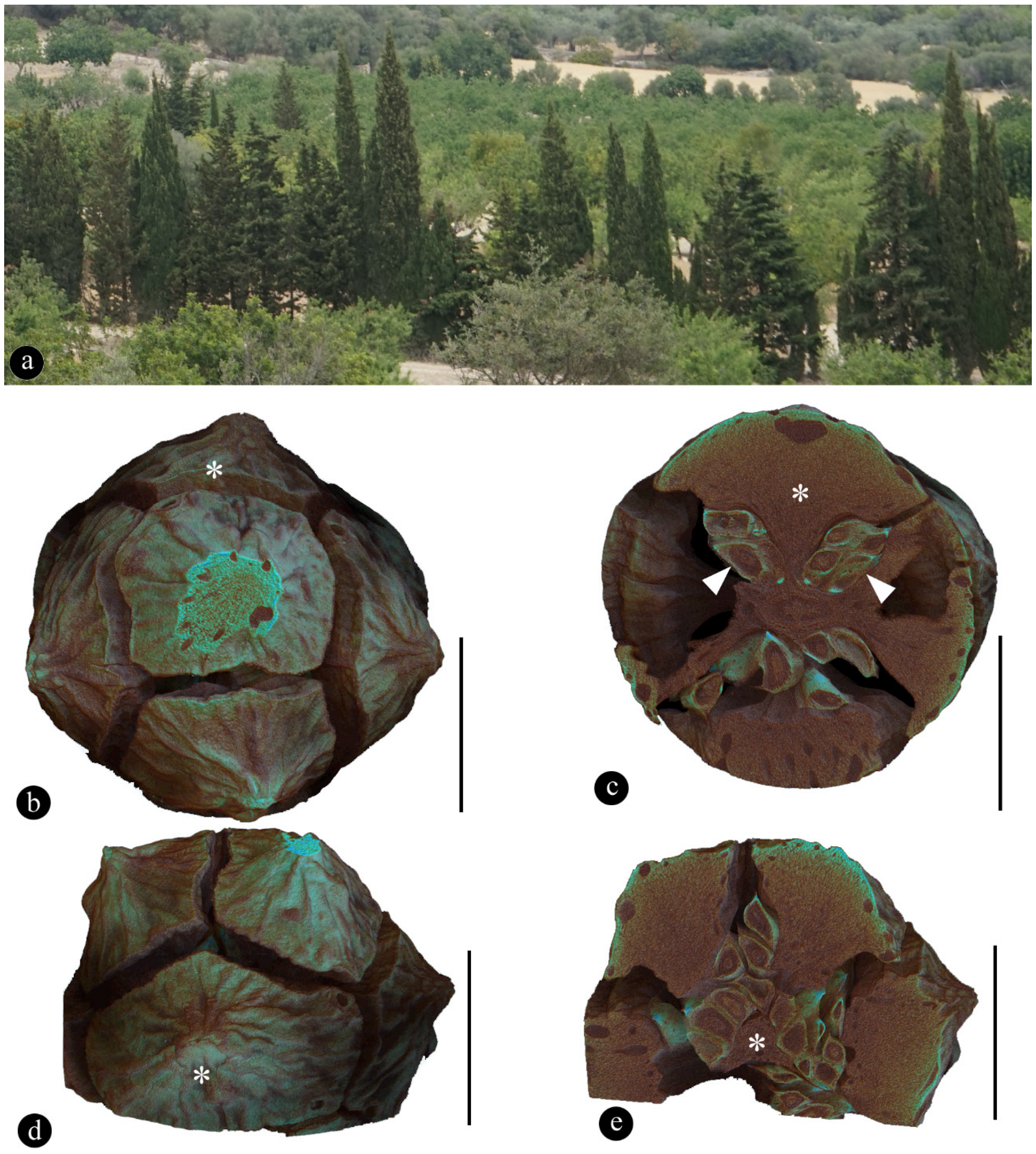The image features a detailed composition with two main sections. The upper section showcases a photograph of an outdoor area densely populated with green trees, potentially lining the side of a road, signifying a natural landscape captured during the daytime. In the bottom left corner of this photograph, the letter 'A' is prominently displayed.

Beneath this top photograph, the image transitions into a grid of four smaller photos or illustrations, each marked with the letters B, C, D, and E in their respective bottom left corners. These four images have a microscopic or cross-sectional quality, characterized by their predominantly brown hue and circular shapes. The texture in these photos is intricate, featuring cracks and irregular polygonal sections, along with some green and dark areas interspersed within the designs. The background of this section is stark white, enhancing the contrast and detail of the observed patterns.